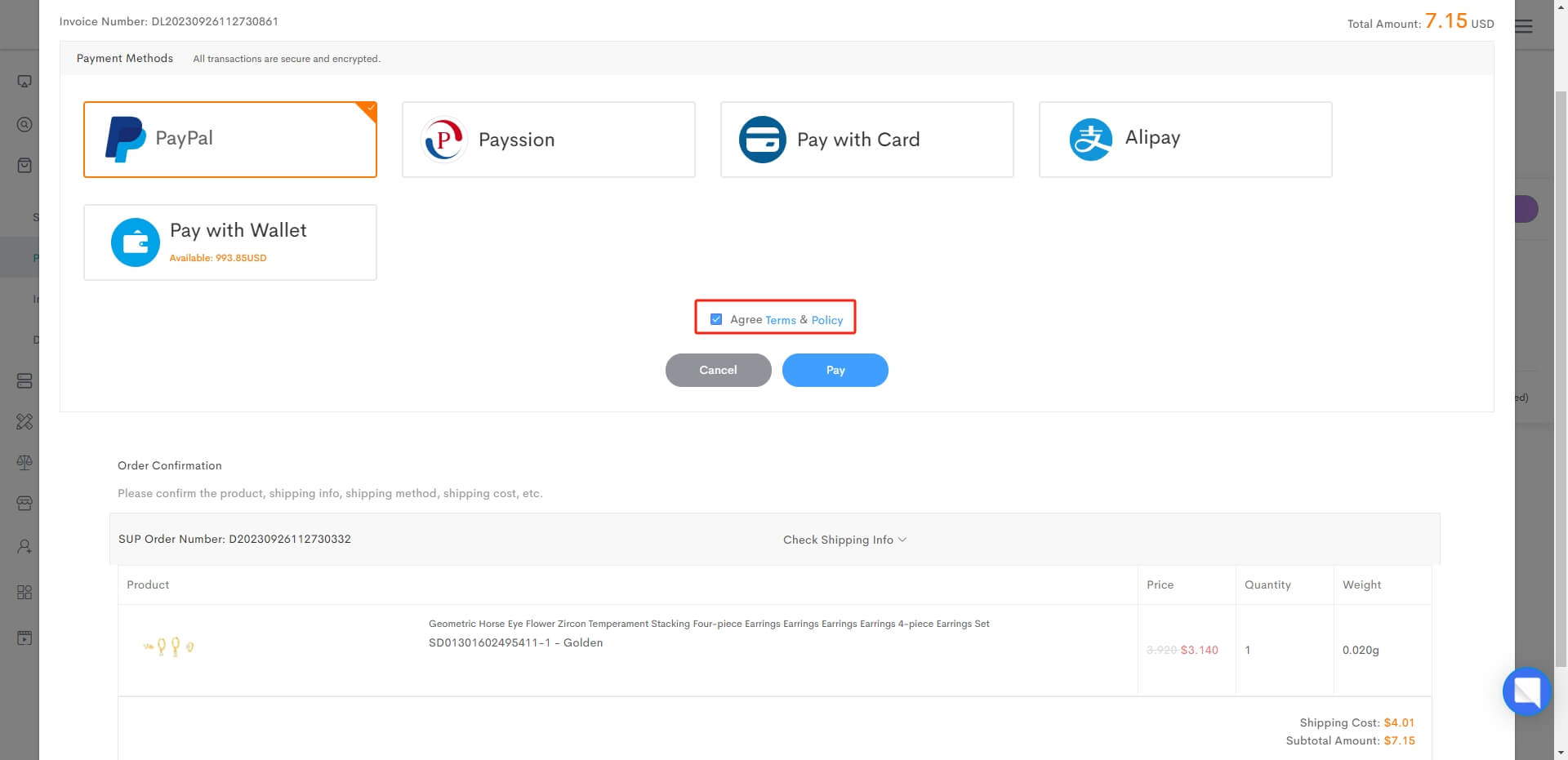The image depicts a detailed screenshot of a website for processing an invoice. The background features both right and left borders in light gray, with the left side housing various navigation tabs, although specific details of these tabs are unclear. The central content is dominated by an interface that appears to be an invoice summary.

On the left side of the invoice, various sections can be observed including a user ID, which could likely be an email address, followed by additional sections that are difficult to read but include recognizable icons such as a YouTube icon and a user ID icon. 

In the middle of the screen, within a very faint gray box, are the words "invoice number," which are not clearly readable due to the small font size. To the right of this box, the total amount due is prominently displayed as $7.15. Below this, another gray box indicates the available payment methods, emphasizing that all transactions are secure and encrypted. The selected payment method is PayPal, with alternative options for payment with a card, Alipay, and a digital wallet also listed.

In the center of the interface, there is a red box with a checkbox that has been selected, indicating agreement to the terms and policy. Directly beneath this are two action buttons labeled "Cancel" and "Pay," with the "Pay" button being highlighted.

Following these buttons is a section for order confirmation, which includes text that appears to request the user to confirm the product details, shipping information, shipping method, and potentially more, although the text is too small to discern clearly.

Further down, the order details section presents a sub-order number and prompts the user to check the shipping info with a dropdown arrow for more details. The product details are displayed next, featuring a small chart that includes an image of the item—likely two wine glasses—though the image and text are significantly small. The chart also lists the price, quantity (1), and the weight of the product.

The final sections of the invoice display the shipping cost, estimated to be approximately $4.91, and the subtotal amount of $7.15.